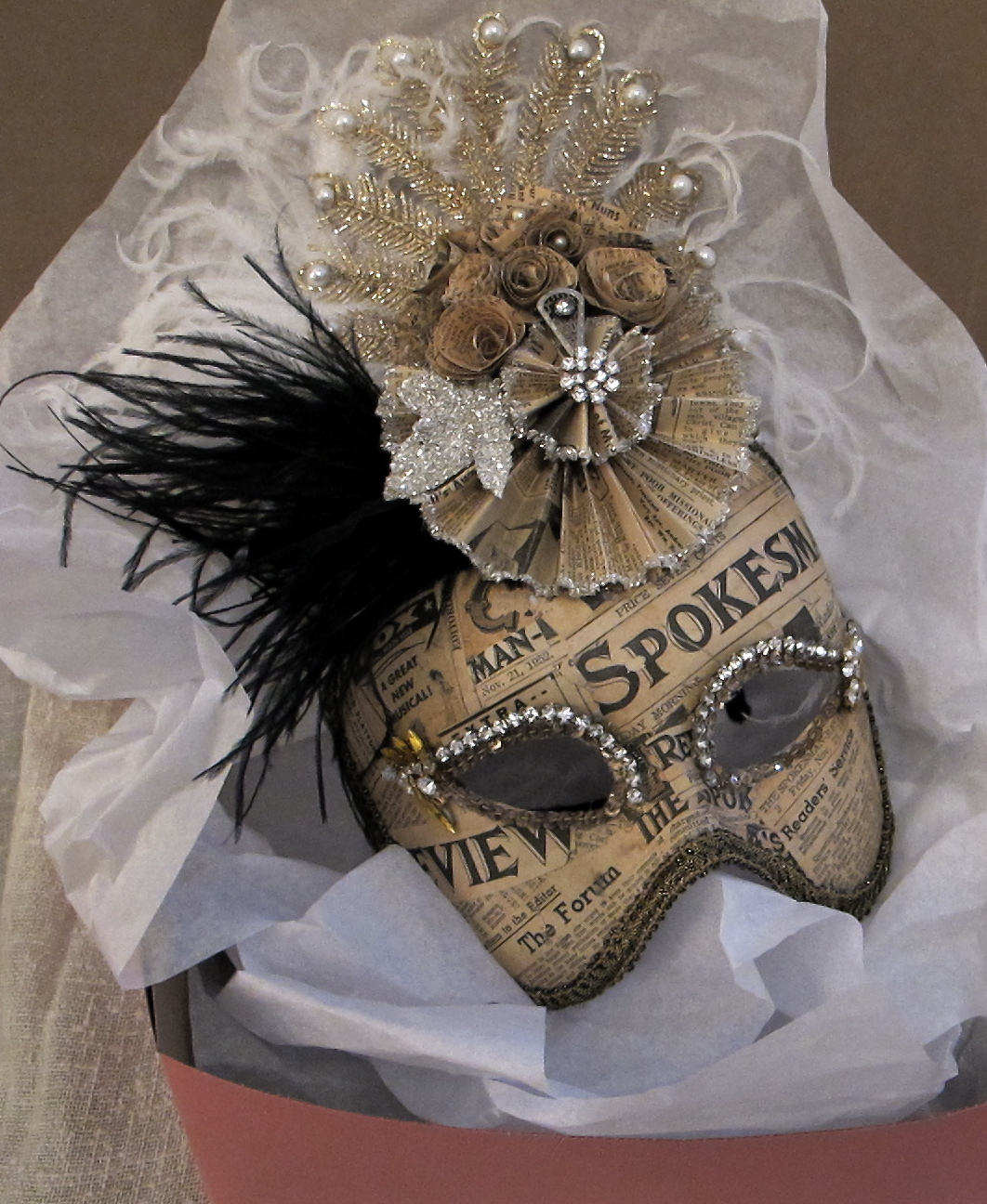The image captures a detailed close-up of a newspaper-decoupage Mardi Gras-style mask adorned with various intricate elements. The mask itself, crafted from old newspaper clippings, prominently features the word "SPOKEISM" on the forehead and has other text fragments like "Man A" and "REVIEW" visible as part of its design. The eye cutouts are bordered with glimmering diamond-like rhinestones, with golden accents at the corners of the eyes. Above the mask, presiding like a headpiece, is a decorative corsage made from beige and gray newspaper, mimicking flowers and embellished with interspersed rhinestones. Golden frills resembling pine needles sprout from this floral arrangement, each tipped with circular gray beads. To the left (the right side for an observer) of the mask, wispy black feathers fan out, adding an elegant flourish. The entire assemblage is nestled inside a red box lined with white tissue paper, and some muslin pieces can be discerned at the bottom left, contributing to the textured background. Additionally, a pair of diamond-lined glasses, seemingly without a visible joiner or with a small string, rests atop the mask, further captivating the viewer's eye with its blend of materials and craftsmanship.